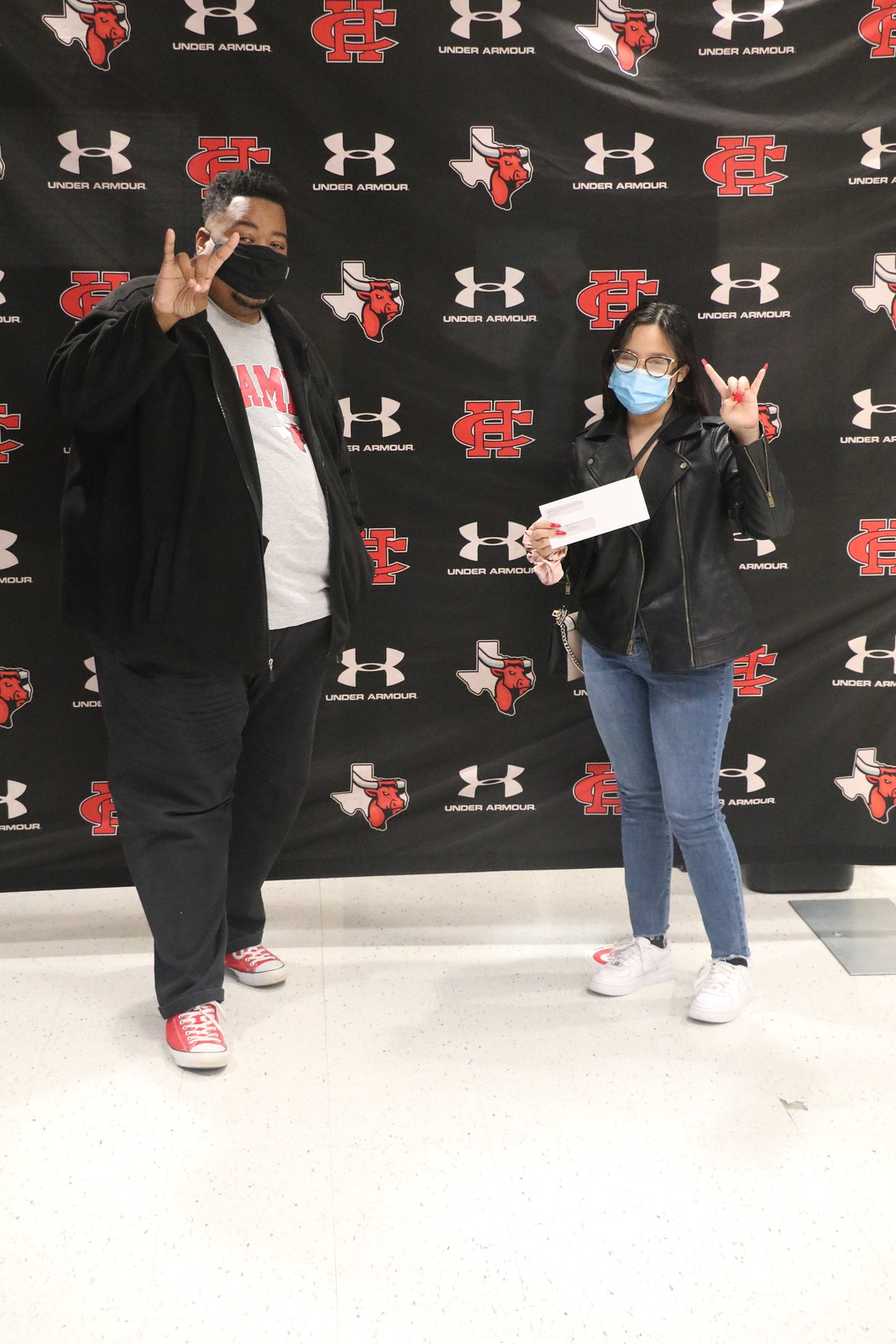This is a full-color photograph taken indoors at a Texas-themed event sponsored by Under Armour. The backdrop features a large red Brahma bull and a college logo with intertwined letters C and H. The image has a peculiar lens effect that makes the two individuals in the frame appear shorter and wider than usual. 

On the left stands an African American man wearing a black mask, black jacket, white shirt with pink lettering, dark grey pants, and red shoes. He is gesturing with the "horns up" hand sign. To the right is an Asian woman with black hair and glasses, sporting a black leather jacket with zippers, blue jeans, white shoes, and a black and grey purse slung over her shoulder. She too wears a black COVID mask and long red fingernails. She holds an envelope and makes a similar "horns up" gesture as the man. They are standing on a white floor with flecks, against the marketing banner bearing the Under Armour logo, Texas imagery, and the C and H logo.